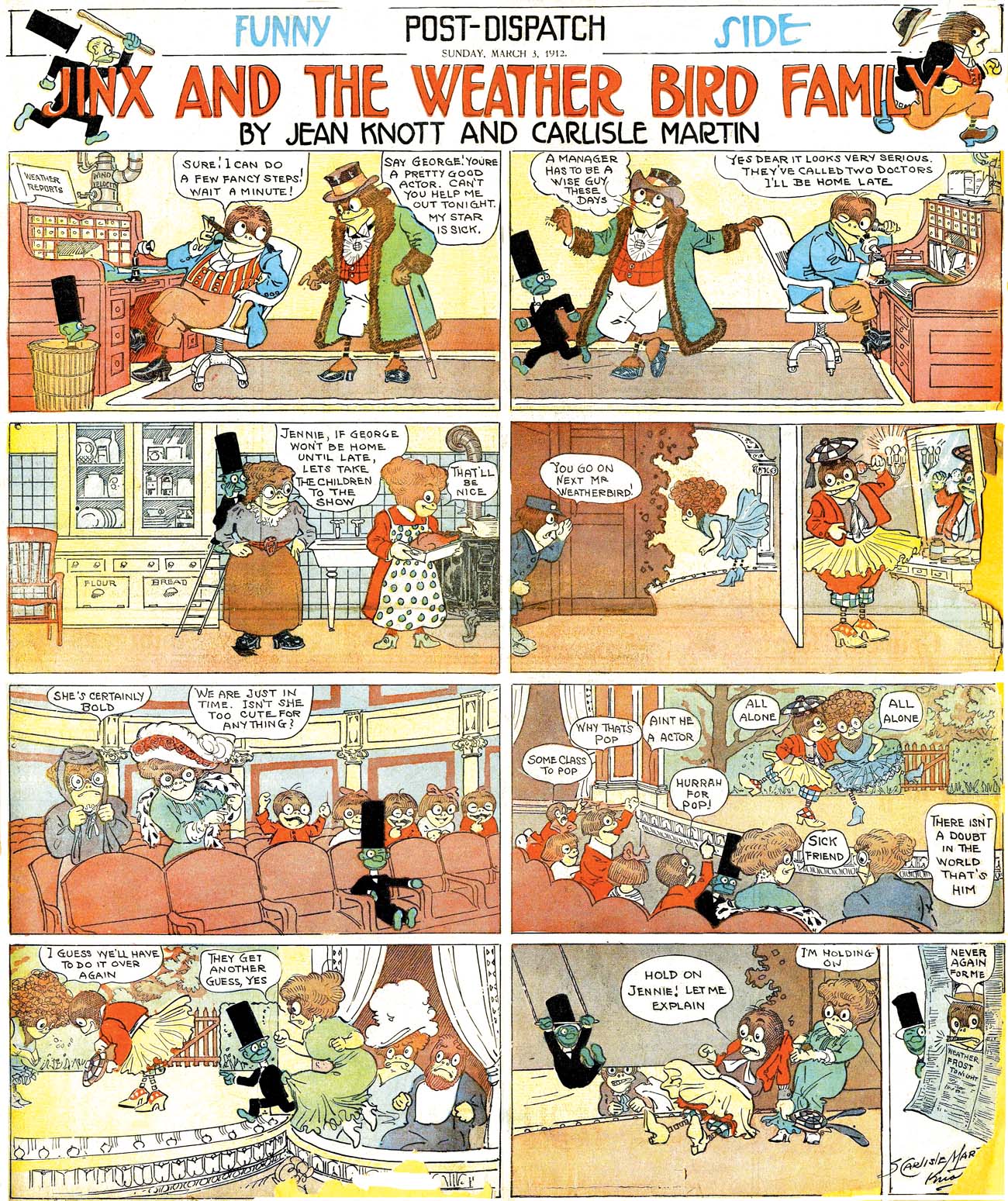This detailed vintage full-page cartoon, titled "Jinxed and the Weatherbird Family" by Jean Knott and Carlisle Martin, appeared in the Post-Dispatch on Sunday, March 1st. The title is notably rendered in red. Featuring a sequence of eight panels, the comic strip includes humorous scenarios depicted under the heading "Funny Side." The panels illustrate two primary frog characters, anthropomorphized with human attire. One frog wears a green coat with a red vest, white pants, and blue shoes, while the other is dressed in a blue coat, a striped vest with reds and whites, brown pants, and black shoes. 

Throughout the scenes, which include an office, kitchen, and theater, the frogs engage in various activities. Notably, one frog is shown sitting at a piano while the other approaches with a cane. The storyline transitions to them attending a play, characterized by an ornate stage with red seats and white curtains. The art showcases a range of colors from light red to tan, light blue, and green, contributing to its old-timey charm with vintage elements such as hats, canes, and fur-lined coats. Each of the four strips contains two panels, each contributing to the unfolding of a continuous humorous narrative.